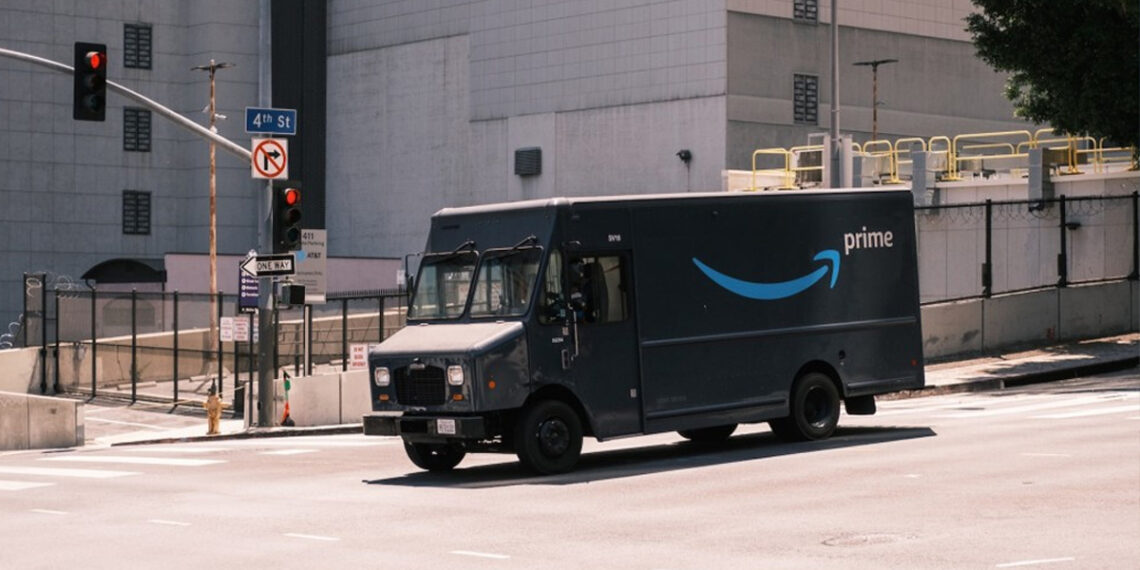In this detailed urban scene, an Amazon Prime truck prominently features the unmistakable blue arrow and "Prime" branding as it heads down a one-way street named 4th Street. The street is marked by a noticeable incline, indicating the truck is descending. It appears the truck is departing from or near a facility that could be a warehouse, characterized by an aging, plain white building with grayish, slightly dirty areas. Behind the truck, a black barbed wire fence hints at a secure perimeter, although it's unclear if it belongs to a prison or another type of warehouse.

A red stoplight looms above the scene, enforcing a momentary pause. Various directional signs populate the area, including one indicating a restriction on turning. A fire hydrant sits at the street corner, accompanied by a large pole displaying multiple signs, including the street name. Despite the Amazon truck’s prominent position in the frame, the driver appears absent or too short to be visible, leaving it ambiguous whether the truck is parked or in motion.